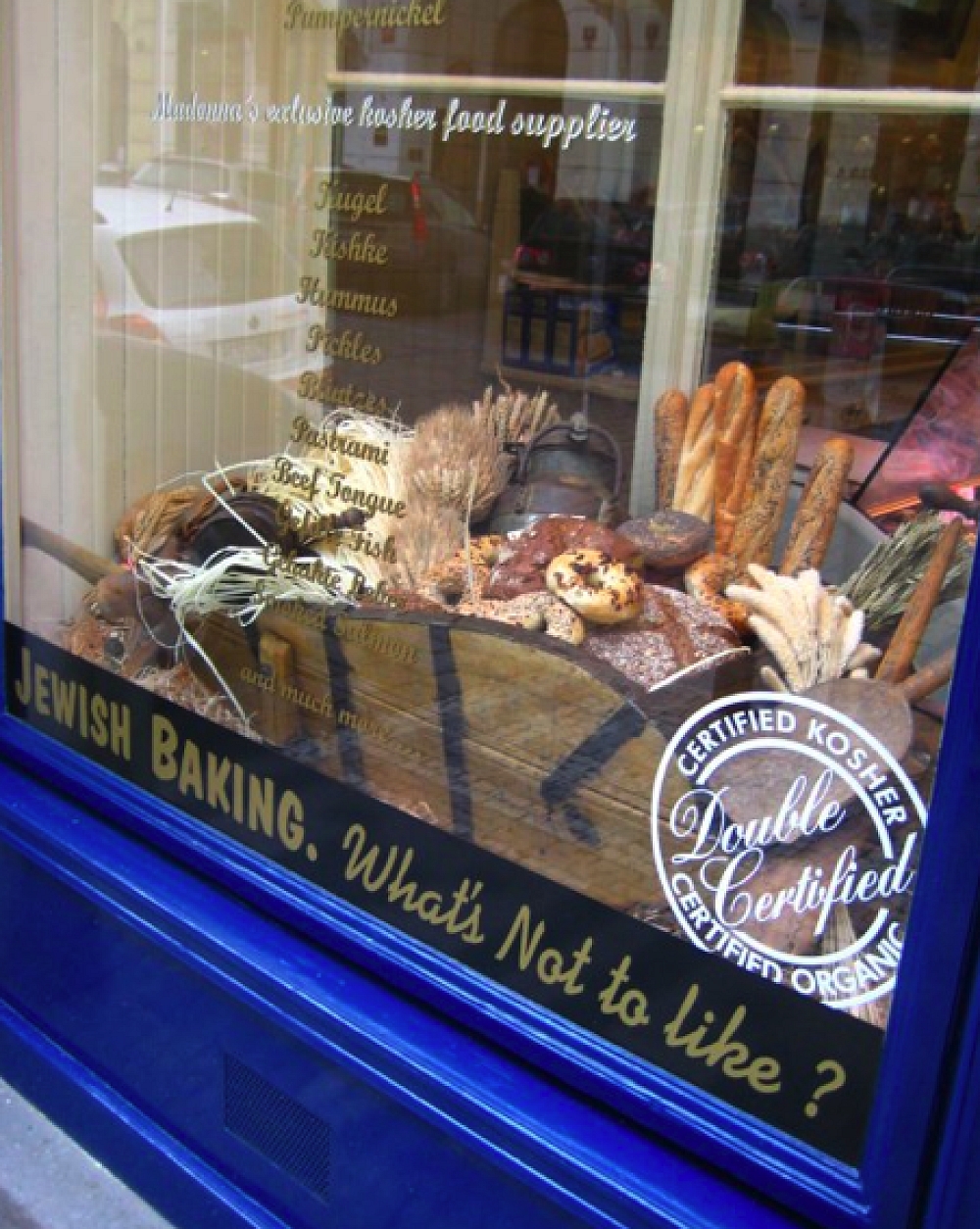This photograph captures the storefront window of Madonna's exclusive kosher bakery. The window, elegantly framed by a rich, royal blue trim, offers a view into the bakery with a vibrant display of various breads. A black banner at the bottom of the window bears the gold cursive text, "Jewish baking. What's not to like?" In the bottom right corner, there's a white circular stamp declaring "Certified Kosher, Double Certified, Certified Organic." The display inside showcases an assortment of fresh baked goods, including upright baguettes, colorful bagels with diverse toppings, and round loaves of bread. Some bakery items are arranged in wooden baskets and on a table, creating an inviting scene. The glass window also reflects the morning light and the outside environment, including a white car and adjacent buildings, adding depth to the composition.